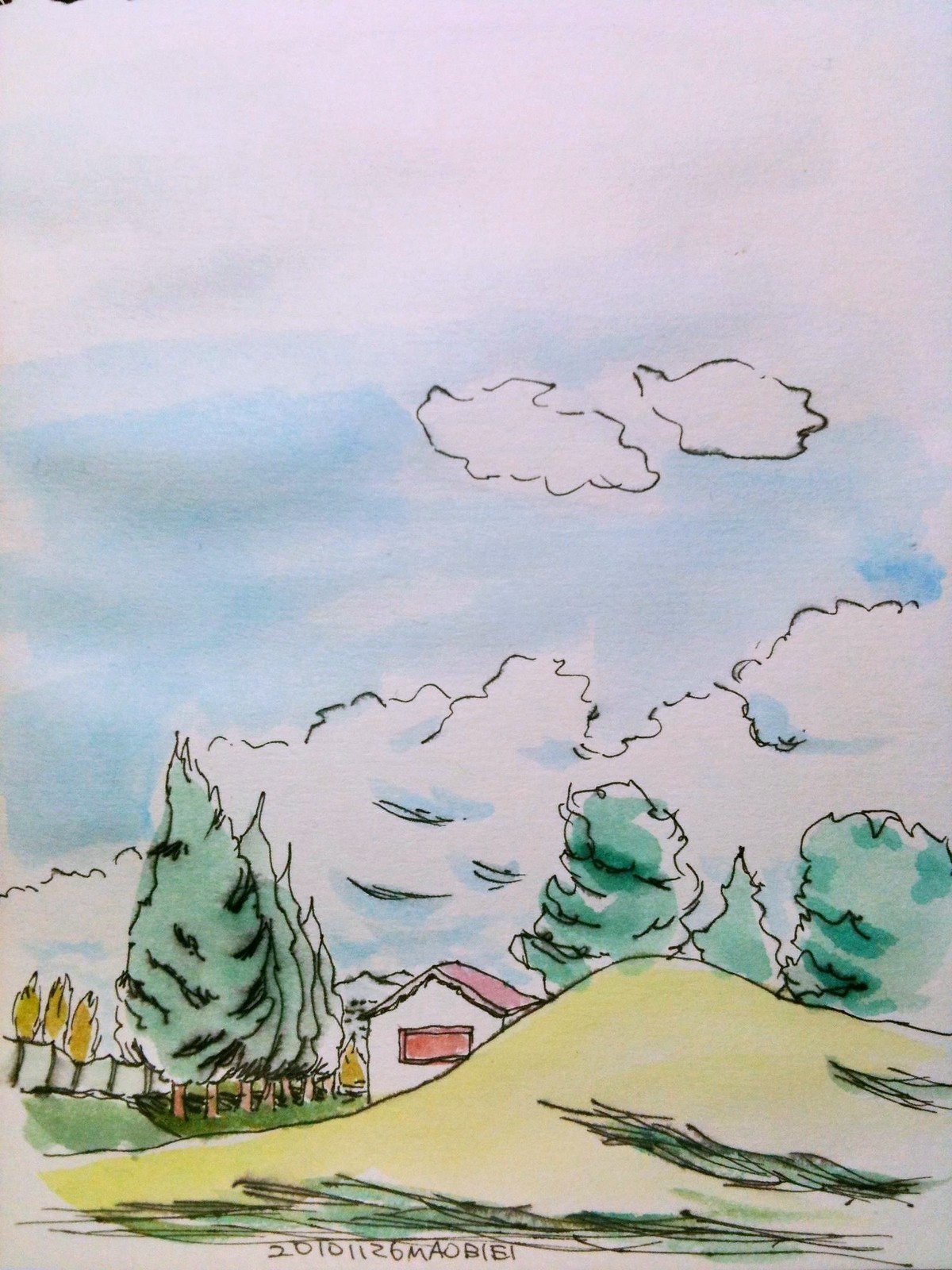This watercolor painting is presented without a frame, and is more vertical in orientation. The composition features a serene sky with two distinct free-floating clouds outlined in black, set against a backdrop of varying shades of blue. Below these, a continuous line of additional clouds stretches horizontally with undulating peaks and valleys, ascending from left to right across the canvas.

In the middle ground, a grove of green trees, interspersed with a few smaller yellow ones to the left, appears to be swaying gently in the wind. Nestled amid these trees is a charming, tiny white house adorned with a pink roof and an orange window.

In the foreground, a hill rises gently to the right of the center, providing a beautiful base that anchors the entire scene. At the very bottom of the painting, an alphanumeric string is inscribed, though its significance remains unclear. Nonetheless, these details underscore the meticulous and delicate nature of this watercolor artwork.